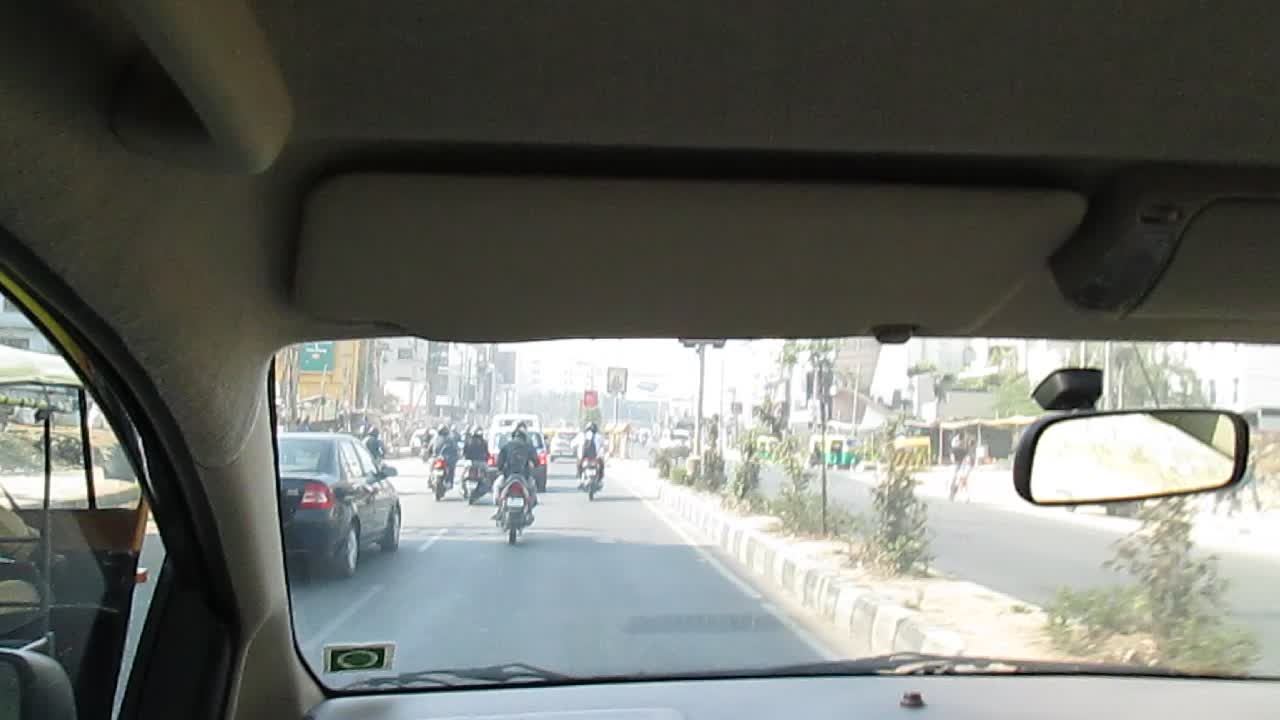A detailed caption for the image could be:

"The photograph captures the view from the driver's seat of a car. Visible in the right side of the image is the rearview mirror, confirming it was taken from the driver’s perspective. The black windshield wipers are apparent on the gray dashboard, with the top of the car showing a light gray or white color. To the left of the driver's position is a black sedan. Central to the image is a group of motorcyclists, appearing to ride black motorcycles. They are positioned behind several cars at a red traffic light, indicating they are stopping in traffic. The road, made of gray pavement, stretches ahead under the clear, daytime sky."